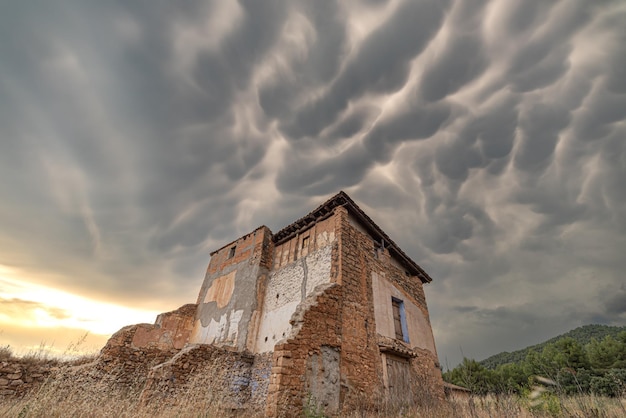The image is a color photograph capturing an ominous and tumultuous sky, dominated by gray clouds that resemble mountain ridges, with the hint of sunnier skies peeking through in the bottom left corner. The foreground features a weathered, dilapidated stone structure, possibly the ruins of a castle or old building. The stacked stonework has heavily deteriorated, revealing the gray and white cement and mortar beneath, though the roof remarkably remains intact. The structure includes a plank wood door on hinges and a framed window above it. Surrounding the structure are tall, wheat-like grasses in a brown and yellow hue. In the distance on the right lower side of the photograph, a green hill or mountain can be seen, blanketed in dense trees. Behind the ruin is a stone wall running parallel to the building, adding to the scene's rustic charm. The overall mood is heightened by the stormy, thick cloud cover that threatens an impending storm.